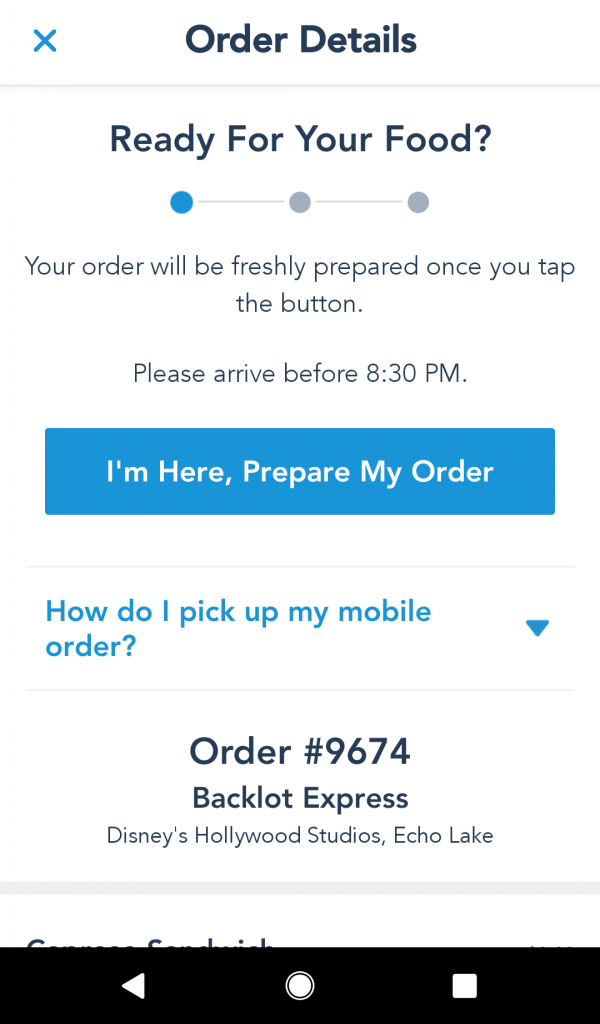Screenshot of a food order status from a mobile app. At the top, the header reads, "Order Details." Below that, it states, "Ready for your food," accompanied by a progress line with three circles, the first of which is highlighted in blue, indicating the current status. The text informs the user, "Your order will be freshly prepared once you tap the button." Additionally, it includes a reminder, "Please arrive before 8:30 PM."

There is a prominent blue rectangular button labeled, "I'm here, prepare my order," for the user to tap upon their arrival. At the bottom, a link is provided with the query, "How do I pick up my mobile order?" which can be expanded via a dropdown menu for further instructions. The screenshot also shows the order number, "#9674," along with the location details: "Backlot Express, Disney's Hollywood Studios, Echo Lake."